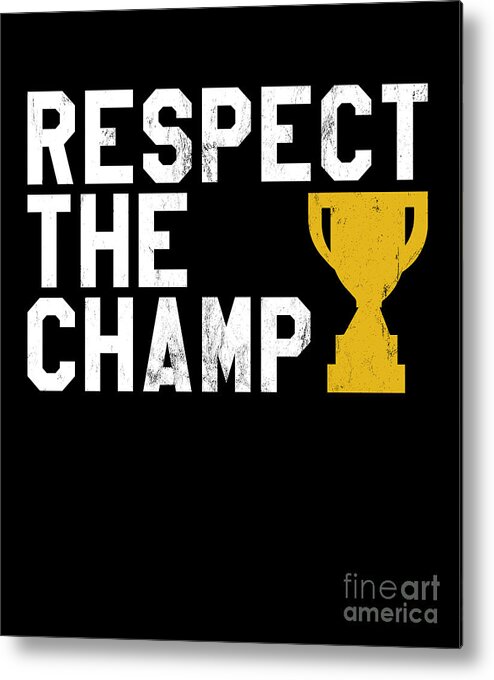The image depicts a detailed painting or poster that almost has the dimensions of a slightly wider book cover. It hangs on a wall, casting a shadow that emphasizes its presence. The artwork features prominent white text against a black background, arranged in three rows, stating "RESPECT," "THE," and "CHAMP." Notably, this white text is imperfect, with visible black splotches appearing more prominently on letters such as the S, P, and C in "RESPECT" and the A and M in "CHAMP." To the right of the text, there is a golden trophy outlined in a similar imperfect style, with black marks visible on its right side. At the bottom right corner, in gray text, it reads "Fine Art America," suggesting that this piece is a work of fine art rather than a book or album. The overall presentation of the image suggests it could be a poster advertising an art show or paying tribute to a champion.